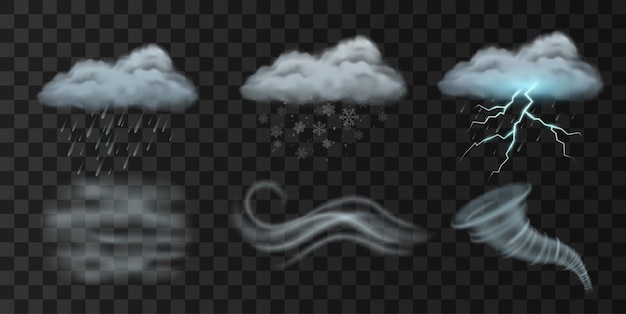The image is a detailed, digitally created drawing set against a checkerboard background of dark gray and black. At the top of the image, there are three identical clouds in shape and size but varying slightly in color. The leftmost cloud has a bluish tint at the bottom and releases raindrops. Beneath it, there's a depiction of a foggy, mist-like phenomenon. The middle cloud is gray and has snowflakes falling underneath it. Below this cloud, there are curvy, horizontal strands representing wind. The rightmost cloud has a much bluer center bottom and emits lightning bolts. Beneath this cloud, a curving tornado shape is illustrated. The scene showcases different weather conditions: rain with mist and fog, snow with wind, and a thunderstorm with lightning and a tornado.